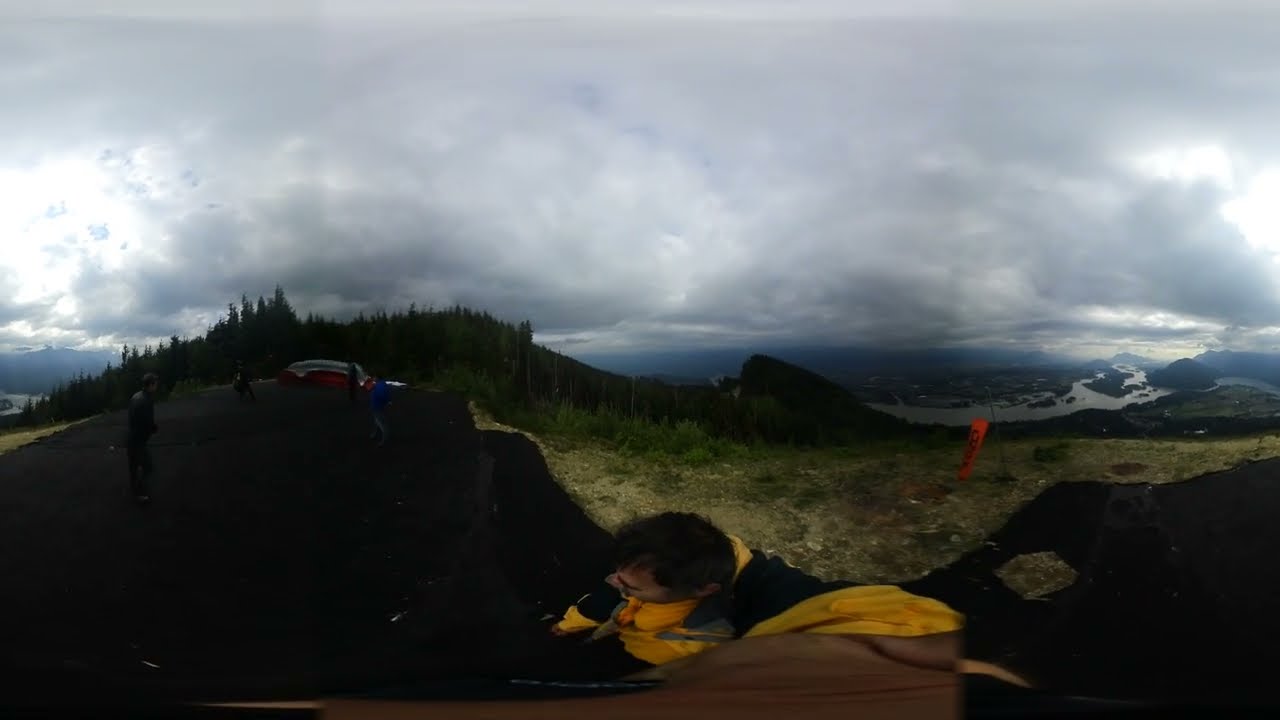The image captures a sweeping, panoramic view from a high vantage point, looking down a hill with a forest and a body of water that appears to be a river. The landscape is framed by hills or possibly mountains in the distance, but thick, low-hanging clouds obscure much of the background. The scene is set on a very cloudy day, with dark gray clouds dominating the sky, punctuated by occasional bright spots on the left and right edges of the frame.

In the foreground, a person with dark hair, wearing a yellow and black outfit, stands prominently. Their arm, clad in yellow, is exaggerated due to the fish-eye lens, and they appear to be holding the camera up. The distorting effect of the 360-degree lens makes close elements appear skewed. Another individual is visible to the left of the person holding the camera, either walking away or gazing at the view. Both figures are positioned on dark, blacktop ground, which may be a roadway or a parking lot.

The terrain immediately in front of the camera holder features dry soil interspersed with grass, transitioning to denser, darker vegetation as the landscape slopes downward. An orange or red flag-like banner lies skewed in the center of the image among the dry soil, partially obscured and unreadable due to the lens distortion. Beyond the forest, the river winds through the land, with hints of a town or city along its banks. The expansive, cloud-heavy sky contributes to the dramatic, moody atmosphere of the scene.